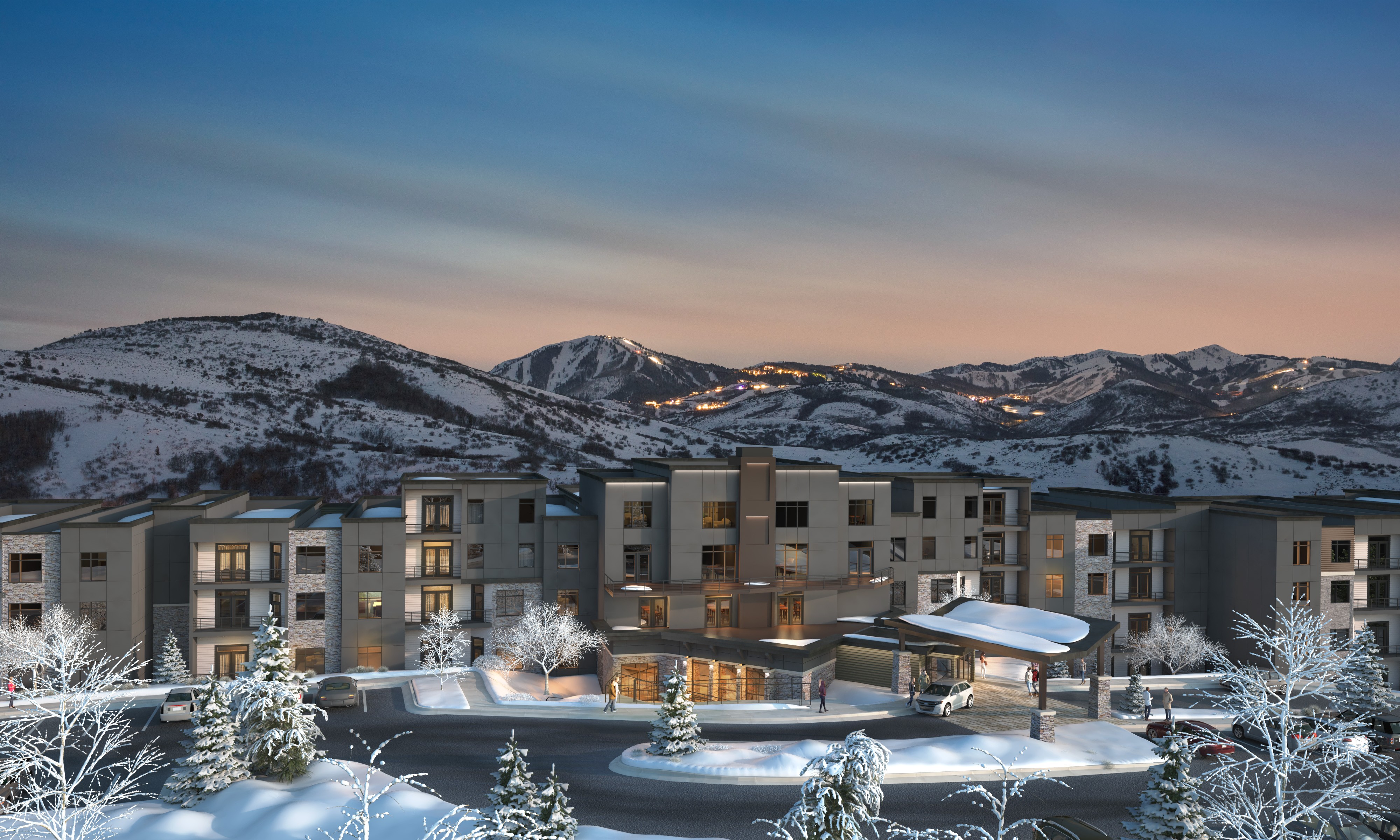The image depicts a serene winter evening scene likely generated by a computer, showcasing a picturesque snow-covered resort. The sky transitions from light blue streaks at the top to a delicate pinkish hue near the horizon, indicating the time is either dawn or dusk. The centerpiece of the scene is a series of half a dozen snow-capped peaks stretching from left to right, possibly skiable mountains with discernible trails.

Below these majestic peaks lies a cluster of buildings with flat roofs, likely made up of hotels or condominiums. These cubic structures exhibit a mix of sizes, rising three or four stories high with some having smaller cubes indented into the larger ones. The main building has an intricate V-shaped portico resembling an open book, under which a car is parked beside an area cleared of snow.

Snow-laden evergreens and deciduous trees add to the idyllic setting, with a cleared black asphalt road winding through the snowy landscape. The lower right corner reveals a parking lot and a small island adorned with a single evergreen. Amber lights glow warmly from inside the lower level of the main building, complementing the hotel-like ambiance.

In the distance, the hills and snow-covered mountains hint at a snow resort, likely meant to cater to skiing enthusiasts, with possible ski chalets or similar structures among the illuminated buildings.